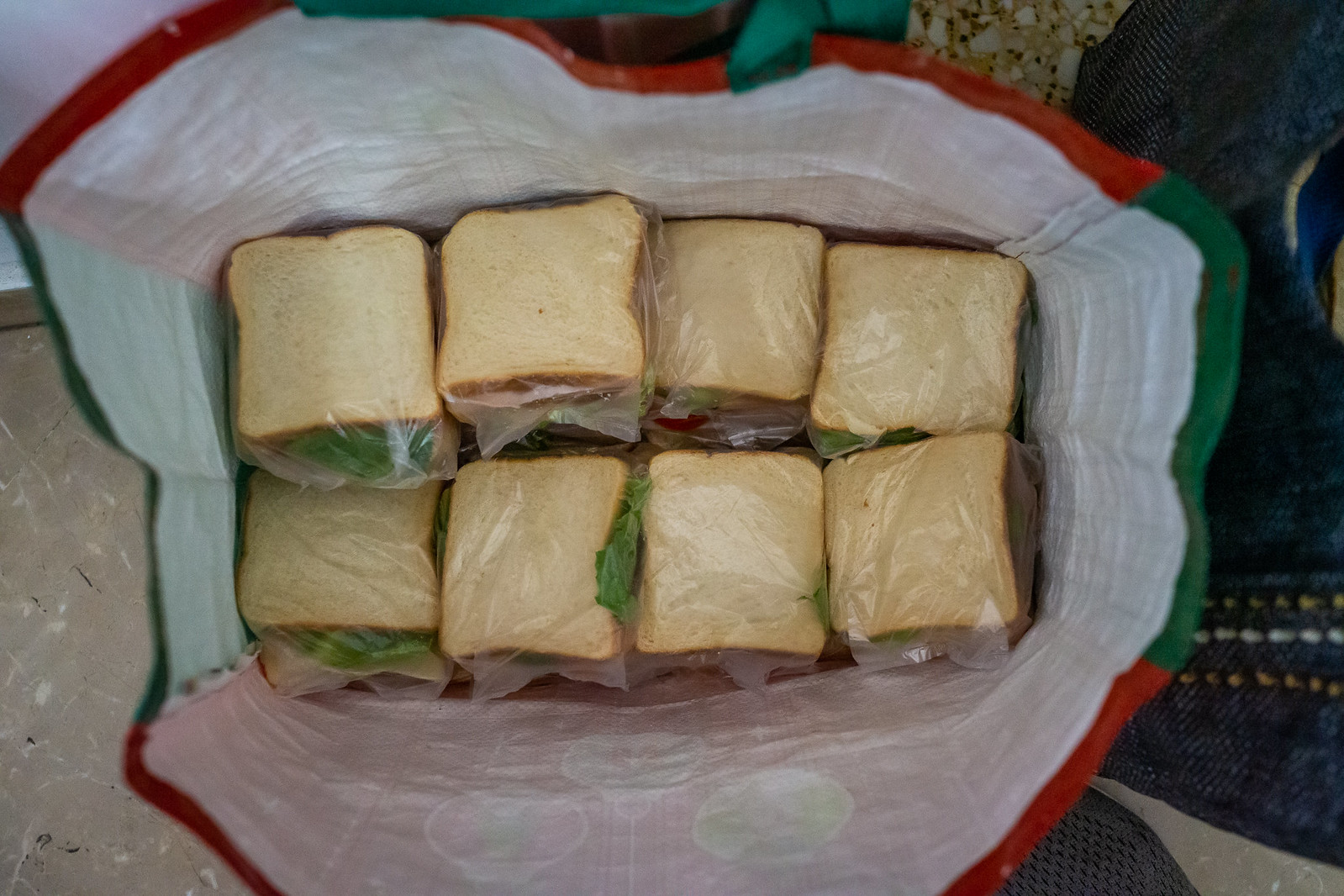This top-down colour photograph captures the interior of a bag-for-life carrier bag, revealing an organized arrangement of eight sandwiches. The bag features a distinctive red circumference at the front and back, green sides, and partially visible green handles extending beyond the frame. The inner lining of the bag is mostly white and slightly translucent, allowing a glimpse of its contents.

The sandwiches, each individually wrapped in clear, polythene-style sandwich bags, are arranged in two rows of four, with white bread visible on their faces. Protruding from the edges of some sandwiches are slices of pink luncheon meat and green leaves, suggesting a filling of ham and lettuce. The photograph is somewhat dimly lit and slightly out of focus, casting shadows on the right where indistinguishable items are barely visible near the edges. The image's top-down perspective and the arrangement of sandwiches imply they are ready for presentation, possibly at a gathering or event.